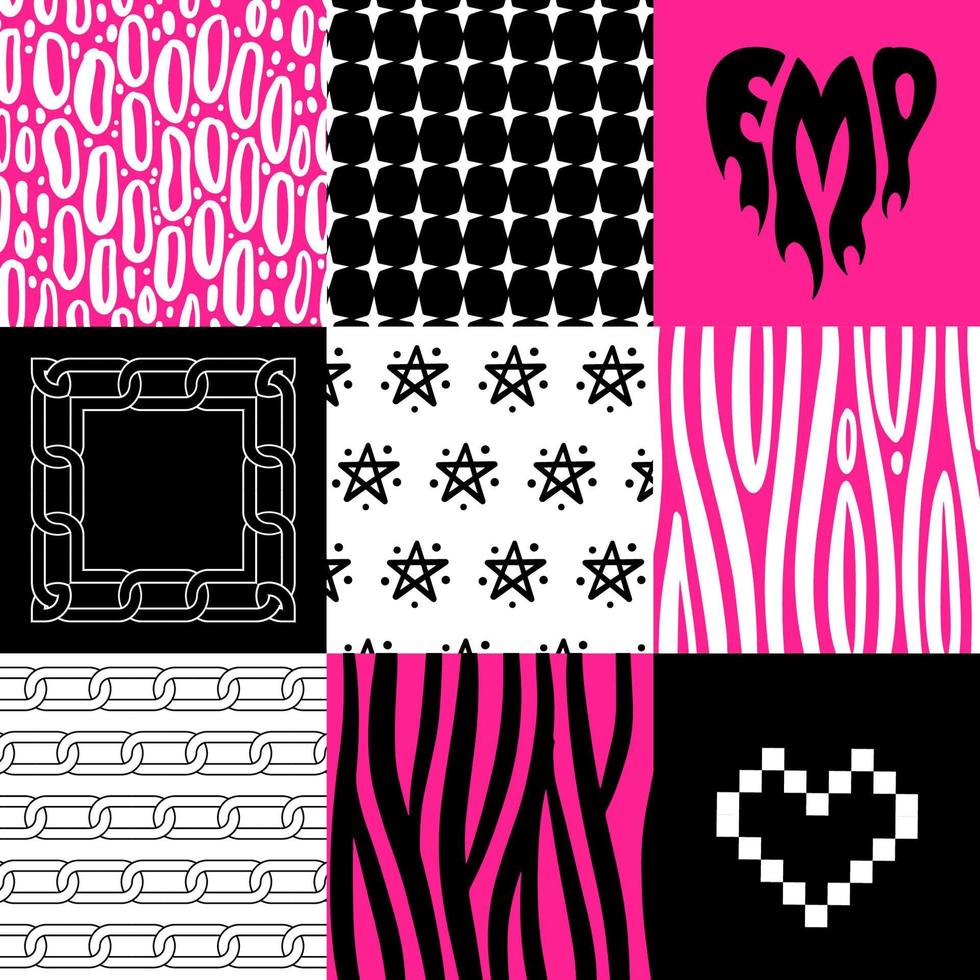The image consists of nine meticulously arranged squares, each showcasing a unique and vibrant abstract design with a prominent palette of bright pink, white, and black. In the top row, from left to right, the first square features a bright pink background adorned with white open ovals. The second square presents a star design created in the negative space of black squares on a white background. The third reveals the bold black letters "EMP" with flames at the bottom on a vivid pink backdrop. 

In the middle row, the left square highlights a black background with a white chain outline encased in a square. The center square displays black stars and dots on a white background. The right square exhibits a bright pink background with dynamic white lines reminiscent of zebra stripes.

The bottom row begins on the left with a white background featuring horizontal chain outlines. The center square continues with a similar zebra stripe design, but this time with black stripes on a bright pink background. The final square on the right showcases a white pixelated heart on a solid black background. This intricate and colorful ensemble creates a cohesive visual mosaic that blends various abstract patterns into a striking composite image.